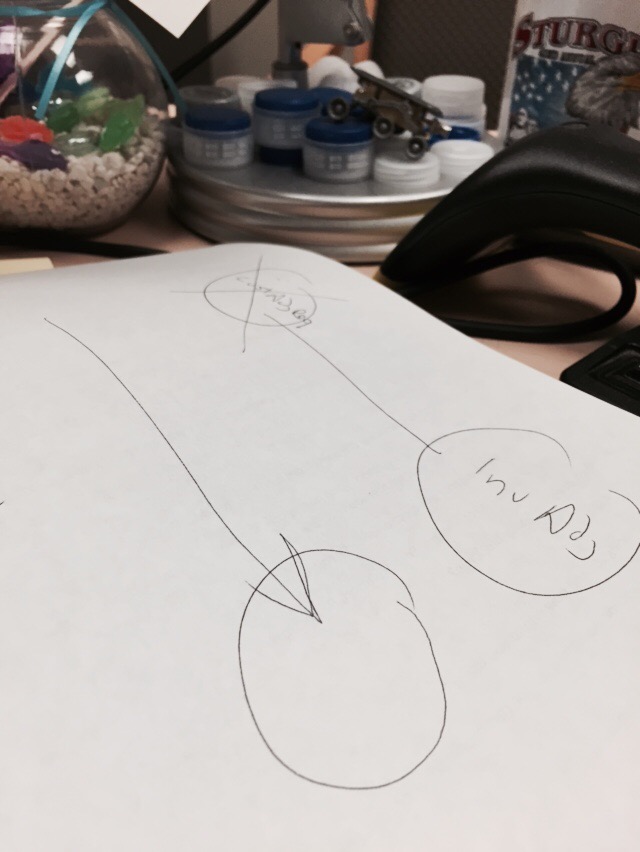On the table, there is a small fishbowl filled with white rocks, a little black fish, and some green leaves. Floating in the bowl are a red object and blue and pink ribbons adorning its exterior. A piece of paper hangs down at the top edge of the image, alongside a black strap rising vertically. To the right of the fishbowl is a stack of three or four white plates, accompanied by several small white jars with blue tops and gray labels. Nearby, there's a toy car or a railroad car in gray. A white bag with red lettering, accented with blue and gray, is also present. Additionally, a black appliance sits on the table next to a piece of white paper featuring a diagram with arrows pointing to circles, with one circle being crossed out and another containing a few letters.